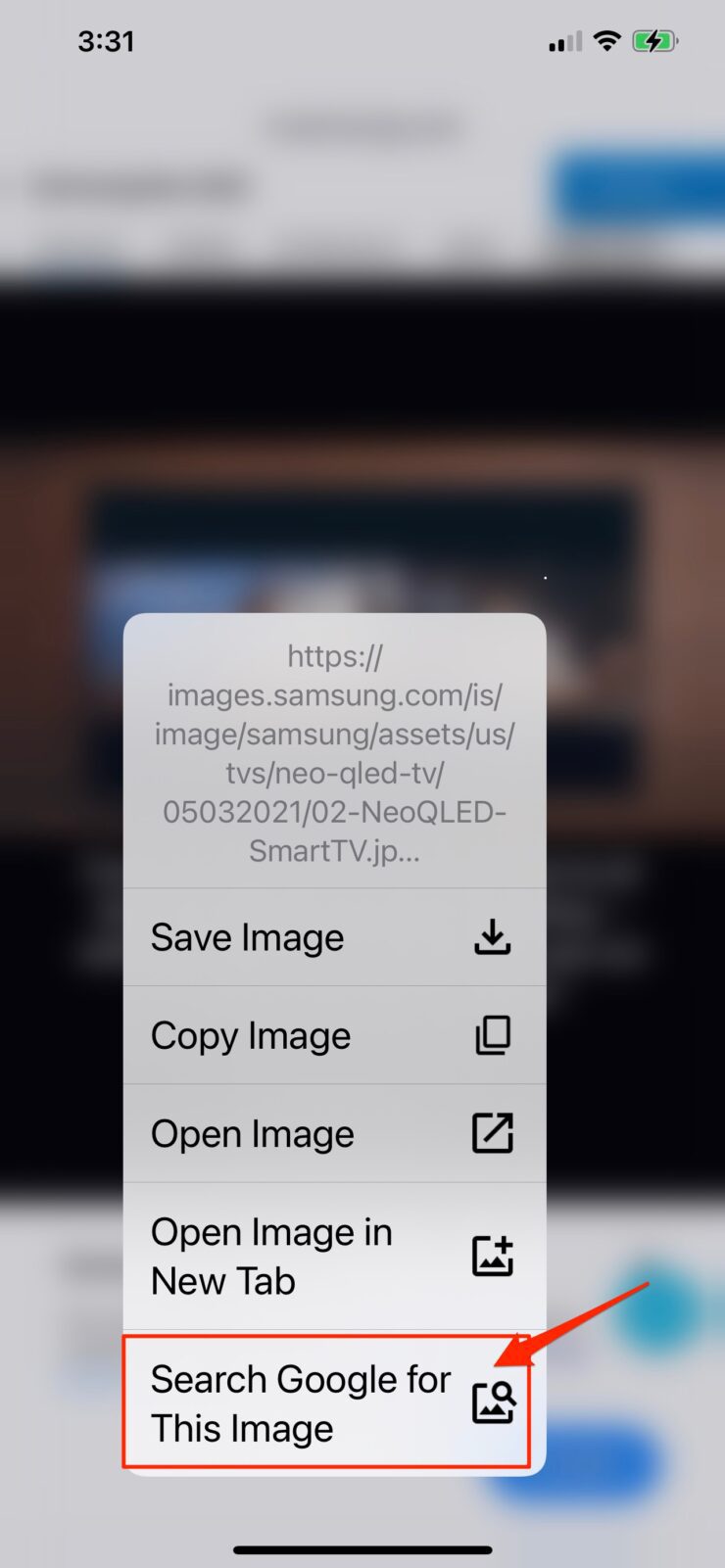This screenshot, captured from a cell phone, depicts a somewhat busy interface with various informational elements. The background of the phone shows a blurry image, which could potentially be an app interface or a webpage, making it difficult to discern precise details. At the top left corner, the time is displayed as 3:31. To the top right, there are indicators for cellular signal strength with two bars, Wi-Fi strength with three bars, and a battery icon filled almost to capacity (between 98-99%), signified by a green icon with a black lightning bolt.

Central to the screenshot is a pop-up menu triggered by a long-press action on an underlying image. The pop-up features a URL starting with "HTTPS://images.samsung.com/" leading to an image of a Neo QLED TV. Below this URL, several actionable tabs are listed: "Save Image," "Copy Image," "Open Image," "Open Image in New Tab," and the fifth option, highlighted with a red rectangular border and red arrow, is "Search Google for this image."

This pop-up indicates the actions available for the long-pressed, blurry background image, suggesting options for manipulating or searching for that image on the device.